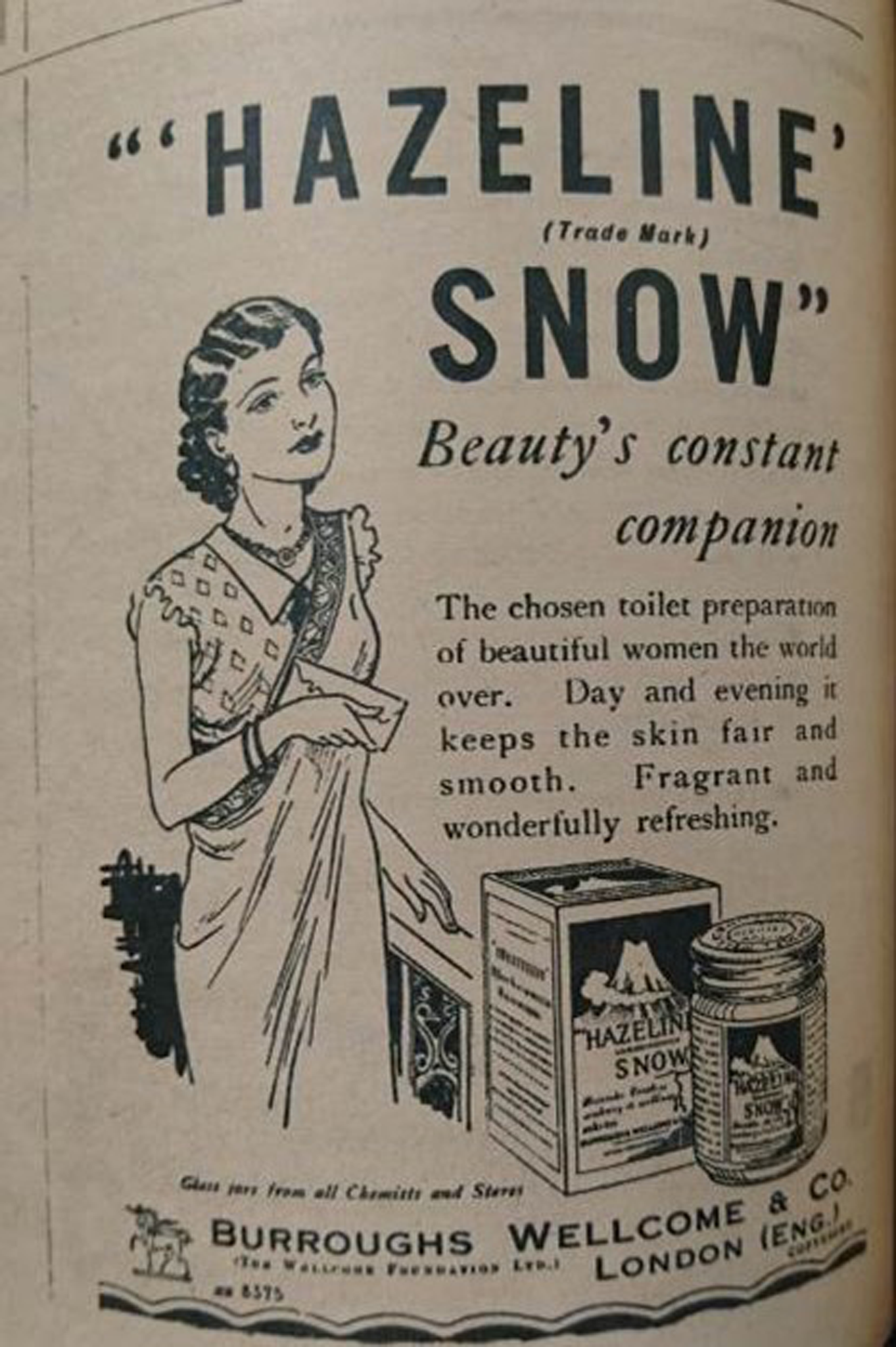The image is a vertical rectangular advertisement or package label for a product called "Hazeline Snow." At the top, in large black letters, it says "Hazeline" with "Snow" in big black letters underneath, followed by "Beauty's Constant Companion" in smaller black letters. Below this, a detailed description reads, "The Chosen Toilet Preparation of Beautiful Women, The World Over. Day and Evening, It Keeps the Skin Fair and Smooth, Fragrant and Wonderfully Refreshing." 

On the left side of the image stands a woman adorned in a fancy dress with a necklace, her hair styled in curls forming lines at the top of her head. She wears two bracelets on her right wrist and holds an envelope in her right hand. Positioned in the bottom right corner are a box and a jar of Hazeline Snow, displaying the emblem "Burroughs Wellcome and Company, London.” The woman and products are hand-drawn, giving the image an old-fashioned, printed appearance in black and off-white tones.